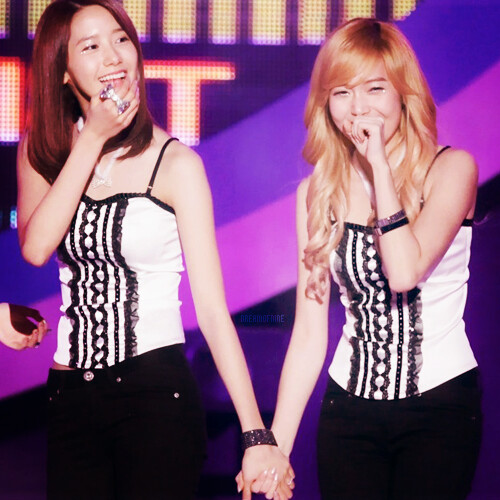The photograph features two young women, seemingly performers, standing close to each other on what appears to be a stage with a digital or graphic background. They are both wearing identical outfits: white tank tops with black straps and intricate black lace trim, paired with black jeans. The woman on the left is slightly taller with dark, reddish-brown hair. She is smiling, holding a large bow-shaped ring on her right hand, which is raised to her mouth, and her left hand is clasping the hand of her companion. She also sports a bracelet on her left wrist. The woman on the right has long, strawberry blonde hair. She is also smiling and has her left hand raised to her mouth. She wears two bracelets. The backdrop features a mix of colors including black, pink, blue, purple, and lavender hues, with some large yellow or orange text, although the text is partially obscured and not fully legible. The overall scene captures a moment of apparent happiness and camaraderie between the two women.